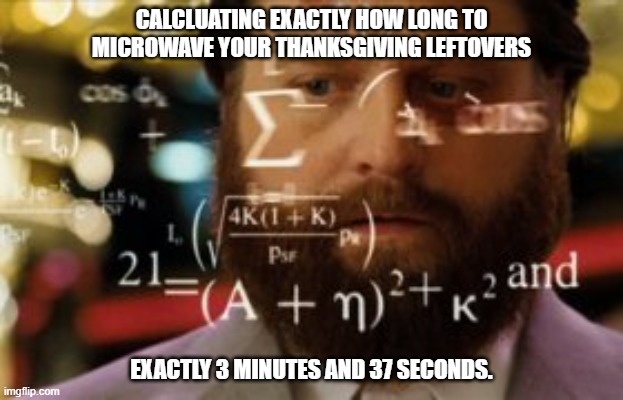The image is a still from the movie *The Hangover*, featuring the character Alan, played by Zach Galifianakis. Alan, a Caucasian man with thick brown hair, a large beard, and a mustache, is dressed in a sharp three-piece suit consisting of a gray jacket, a white dress shirt, and a barely visible gray tie. The background is blurred and brightly lit, suggestive of a bustling casino. Alan appears deep in thought, surrounded by complex mathematical equations floating around him, indicating that he is calculating odds. Overlaid at the top of the image, in white font, are the words: "Calculating exactly how long to microwave your Thanksgiving leftovers." At the bottom, in the same white font, it reads: "Exactly three minutes and 37 seconds." In the bottom-left corner, in small white print, it says "IMGFLIP.com". This humorous image captures the meticulousness of reheating Thanksgiving leftovers to perfection, reflecting on the shared joy and effort of enjoying holiday meals with friends and family.